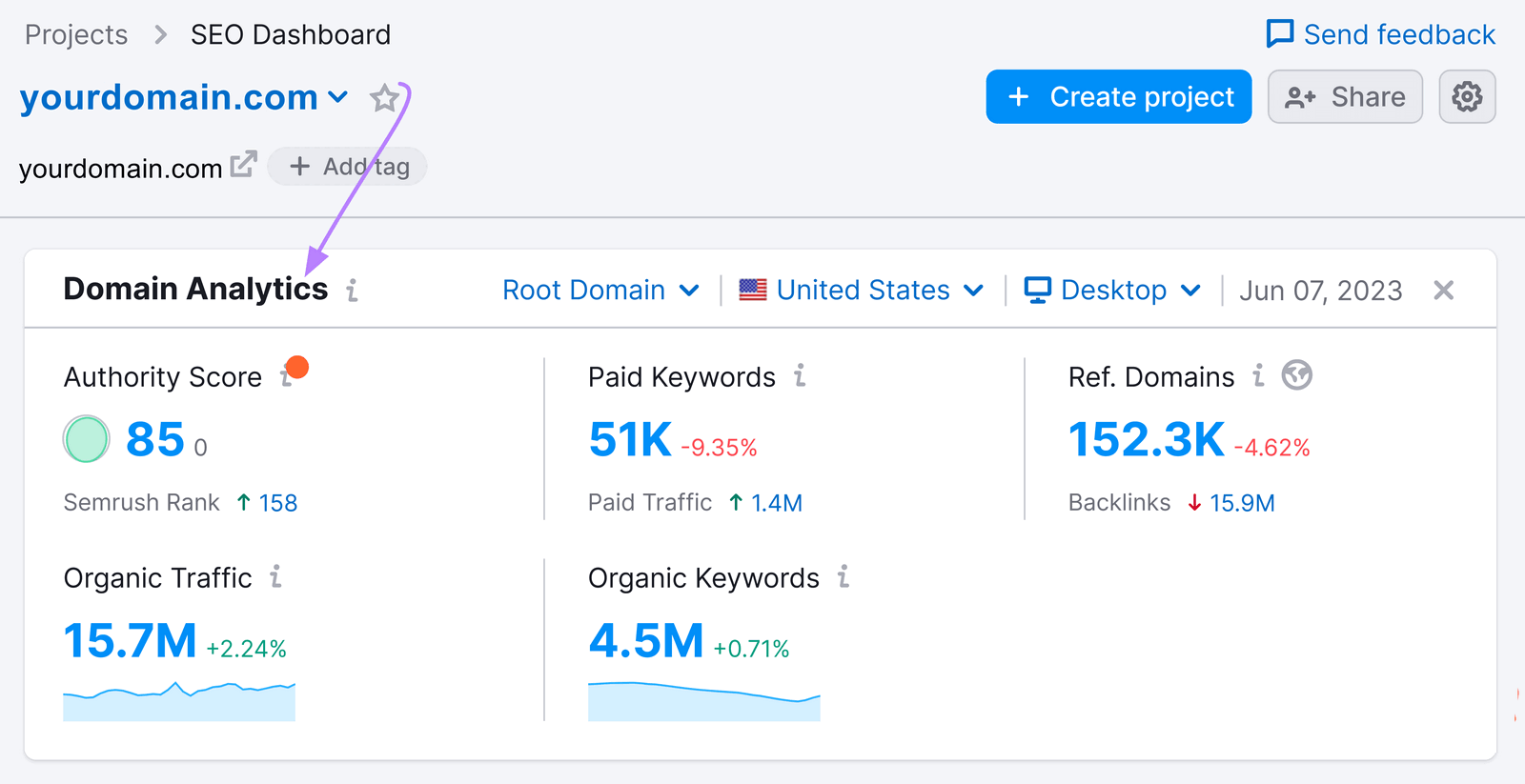This screenshot captures a detailed view of an SEO dashboard from yourdomain.com, emphasizing various metrics and features useful for web management and analytics.

- **Background**: Predominantly light gray or light blue.
- **Header**: 
  - **Top Left**: The word "Projects" followed by a right-pointing caret, indicating a dropdown or expandable menu.
  - **Top Center**: "SEO Dashboard."
  - **Top Right**: "Send Feedback" link.
- **Breadcrumbs**: Slightly underneath the header, it specifies "yourdomain.com" in blue with a dropdown menu beside it, a star icon next to it, pointing towards the next category.
- **Category**: "Domain Analytics" in black on the left.
  - **To the right of this category**: Indicated labels such as:
    - "Root Domain" with a dropdown.
    - "United States" with a dropdown.
    - "Desktop" with a dropdown.
    - "June 7th, 2023" as the selected date.
    - An "X" icon for closing or exiting fullscreen mode.

- **Metrics Section**:
  - **Authority Score**: 
    - Displayed with an orange/red dot.
    - Features a light blue circle highlighting "85" followed by "0".
  - **SEMrush Rank**:
    - An upward-pointing arrow followed by "158."
  - **Organic Traffic**:
    - "15.7M" in blue, indicating a 2.24% increase.
    - A steady trend depicted in a graph.
  - **Paid Keywords**:
    - "51K," showing a 9.35% decrease.
  - **Paid Traffic**:
    - "1.4M," indicating a 1.4% increase.
  - **Organic Keywords**:
    - "4.5M," showing a 0.71% increase.
    - Represented with a bar graph trending downwards.
  - **Referring Domains**:
    - "152.3K," reflecting a 4.62% decrease.
  - **Backlinks**:
    - "15.9M," indicating a decrease (arrow down).

- **Footer Options**:
  - "Create Projects" button with a blue bar.
  - "Share" button.
  - Settings icon on the right.

The layout balances textual information with visual aids like graphs and icons to facilitate comprehensive analysis and quick insights into SEO performance.